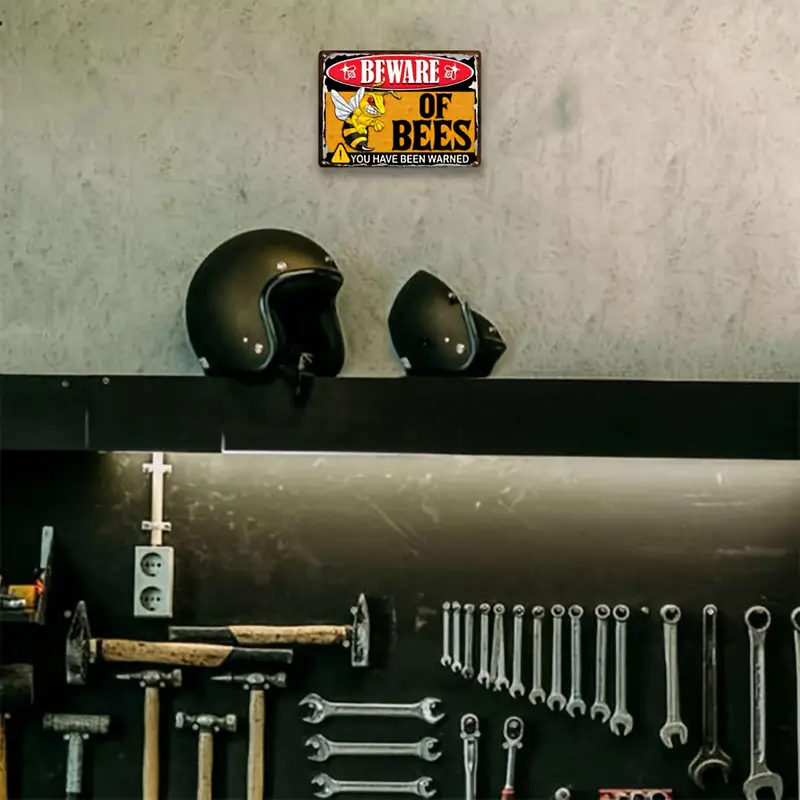In this photograph of a garage workshop, the upper central section of the image features a light gray concrete wall adorned with a striking sign. The sign, displaying a predominately red and yellow design, reads "Beware of Bees" with "Beware" in bold red letters and "of Bees" in solid black text. An intimidating cartoon bee on a yellow background and a cautionary "You have been warned!" are visually prominent below the text. 

Directly beneath the sign, two motorcycle helmets—one larger and one smaller—sit neatly on a black shelf. The shelf stands against a darker slate wall segment, which is systematically equipped with an arsenal of hand tools such as wrenches, hammers, screwdrivers, and chisels, all hanging orderly from hooks. To the left of the organized tool display, an electrical socket box with two outlets is visible, with a wire extending from it, hinting at the functionality and meticulous setup of the workspace. The entire scene is bathed in neutral tones, with the prominent sign providing a vivid splash of color and warning amidst the organized industriousness.